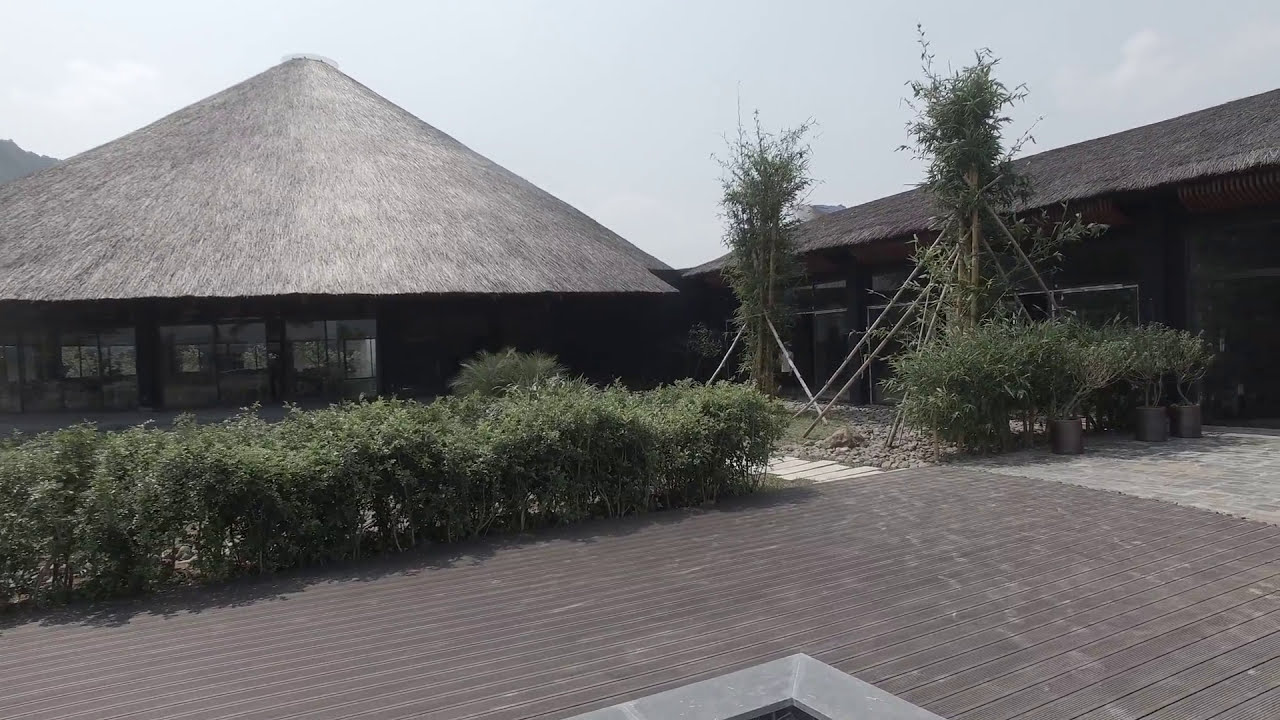The image depicts a brown, tropical-style house with a unique architectural design. The roof, appearing as if it's made from a grassy substance, such as thatch, has a pronounced slope and distinctive lines mimicking grass incorporation. On the left side, the roof is conical, whereas on the right side, it spreads more uniformly but still slopes downward. Directly in front of this section are manicured green shrubs flanked by taller bushes supported by wooden stakes, adding vertical emphasis.

In the foreground, there's a dark wooden walkway seamlessly transitioning into a stone path, creating an inviting entryway lined with lush greenery. This pathway guides towards the brown building, emphasizing the conical roof and its rustic, tropical charm possibly reminiscent of Hawaiian or Asian architecture. The sky above is slightly cloudy and hazy, contributing to a tranquil, subdued atmosphere.